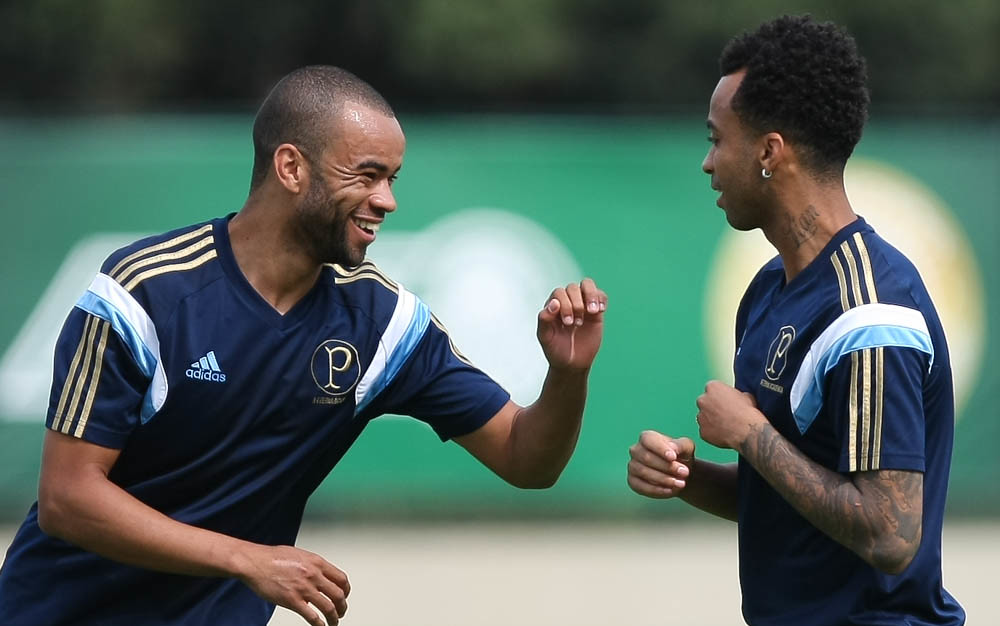In this vibrant photo, two African-American teammates, likely soccer players, are captured in a moment of camaraderie and celebration on the field. Both men are sporting identical blue, short-sleeved jerseys adorned with gold stripes running down the arms, complemented by distinctive white and light blue stitching on the shoulders. Their uniforms feature a gold "P" encircled on the right breast and the Adidas logo in white on the left.

The man on the left, who is bald and clean-shaven, is smiling broadly, as if congratulating his teammate on a great play. The man on the right, sporting short black hair, a silver earring, and tattoos on his neck and arms, is also smiling. His body language suggests he is poised to high-five his teammate.

The background is slightly out of focus but discernible. A green fence with white lettering, possibly signifying the boundaries of the playing field, is visible, along with either stadium stands or shrubbery above it. The ground beneath them is muted, with no clear indication of grass, suggesting perhaps an off-white playing surface. The overall setting radiates the excitement and energy of an outdoor sporting event.